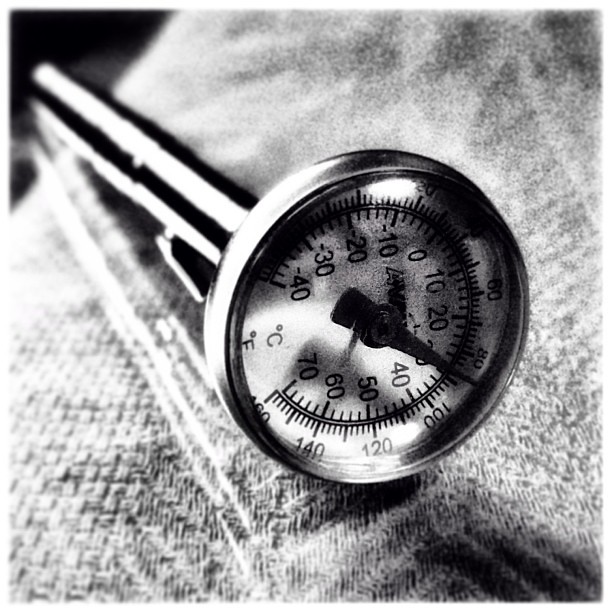A black and white photograph captures a temperature probe or thermometer, mounted on a long cylindrical shaft. The device is positioned at a 45-degree angle, with its large, circular dial and display prominently shown in the lower-right center of the image, facing the viewer. The image backdrop comprises a heavy, woven cloth, adding a textured contrast to the sleek thermometer.

The dial is rotated 90 degrees clockwise so that the scale markings for both Celsius and Fahrenheit are on the left, with mid-range temperatures on the right. The Fahrenheit scale is the outermost, and the needle is pointing to approximately 80 degrees Fahrenheit. Inside the Fahrenheit scale, the Celsius scale is correspondingly displayed. The thermometer appears to be measuring ambient air temperature, registering around 80 degrees Fahrenheit.